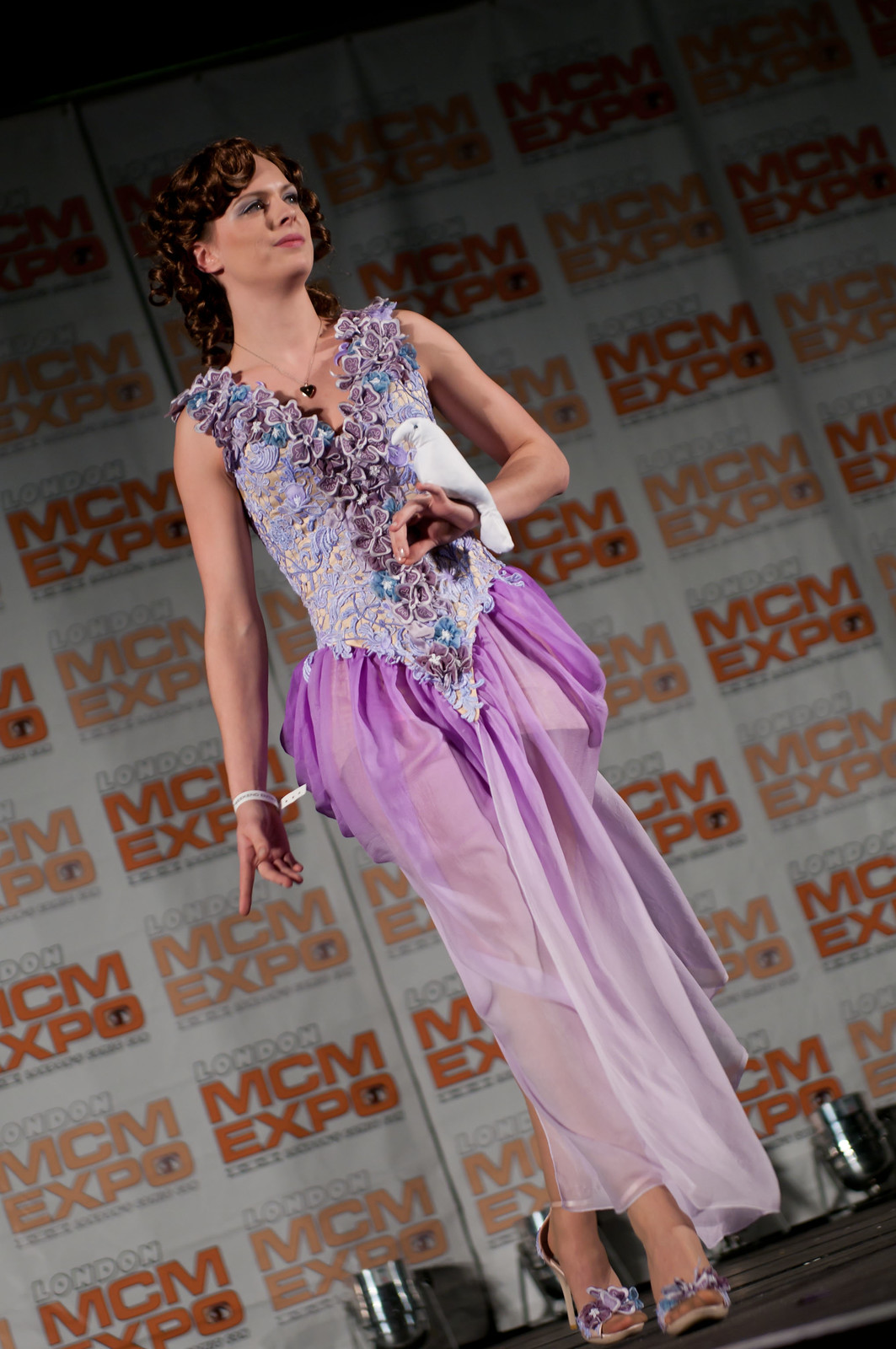The image captures a young, toned Caucasian woman standing on a stage, possibly at a fashion show, photographed at a tilted diagonal angle. She is wearing a long, flowing, sleeveless gown that transitions from medium purple at the top to a lighter shade at the bottom, ending around her ankles, made of see-through chiffon fabric. The gown features a light blue bodice adorned with dark purple lace and floral details that form a V-shape across her shoulders and onto her chest. She has curly, reddish-brown short hair and is accessorized with a heart necklace, high-heeled open-toed shoes that echo the floral design on her bodice. She holds a bird on her left wrist, which she is gently pinching with her fingers, and wears a white band on her right wrist. The stage floor is black, and the backdrop is a white promotional banner with repeated red text that says "London MCM Expo." She is looking out towards the audience with a peculiar expression, her head turned towards the five o'clock position. The angle and lighting give the image a dynamic feel, emphasizing the dramatic setup and her elegant, poised appearance.